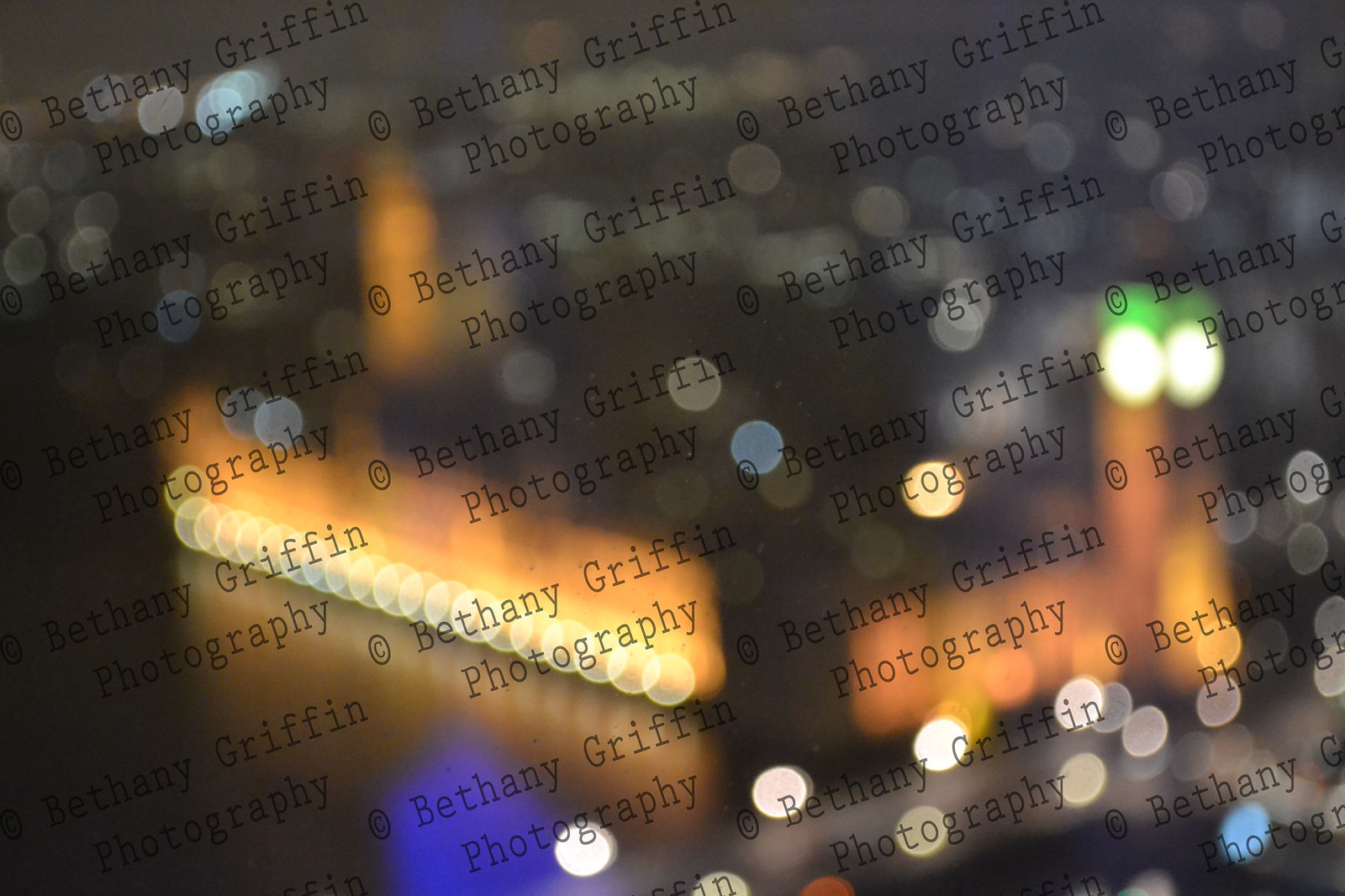The image is a highly out-of-focus photograph, possibly taken in a city street with notable landmarks, but the exact location remains ambiguous due to the blurriness. The out-of-focus effect creates a star-like or bokeh effect with glittery circular lights scattered throughout. Prominent features in the image include a series of rectangular neon signs; one on the center left portion appears orange and yellow, while another similar sign with white and green highlights can be observed on the center right. The photo is extensively watermarked with "copyright Bethany Griffin Photography" in black font, repeated diagonally from the bottom left to the top right corner, with approximately six or seven rows of this text overlaying the image. There are also hints of blue and green tones towards the bottom and the right side of the photograph.